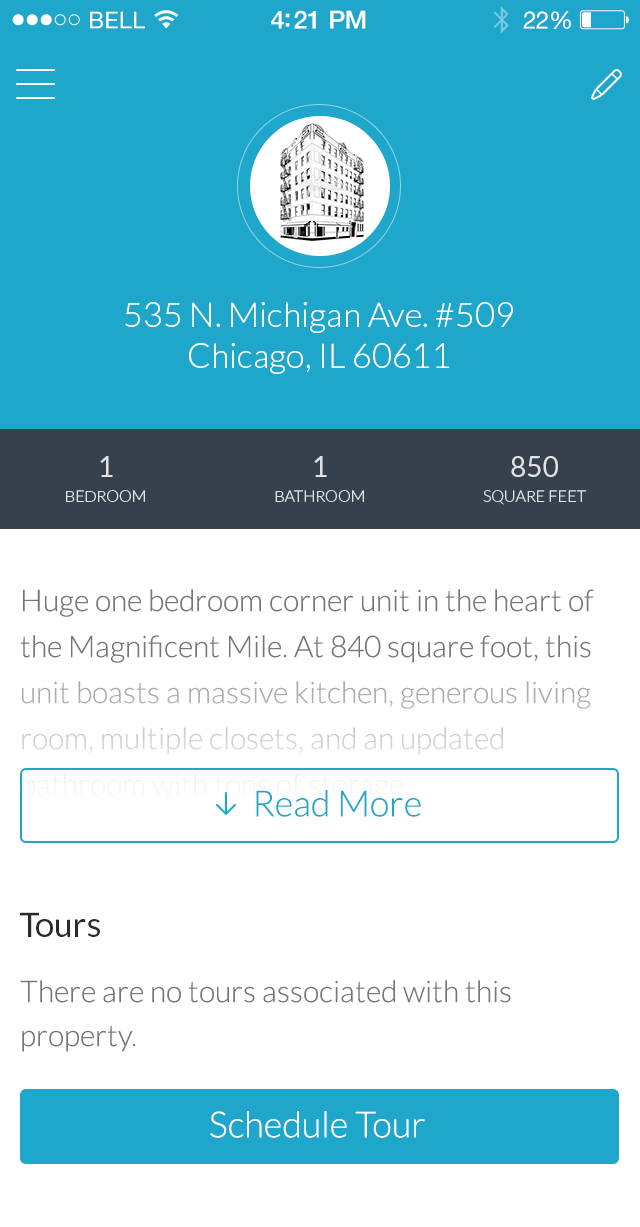This image is a screenshot from a smartphone, capturing a detailed real estate listing. 

**Top Section:**
- The upper third of the image features a beautiful sky blue background.
- On the upper left, "Bell" is displayed, accompanied by three white dots and two outlined circles indicating signal strength.
- To the right, the Wi-Fi icon is visible.
- In the center, the time is shown in white font as "4:21 p.m."
- On the upper right, the battery icon indicates a 22% charge.

**Middle Section:**
- A white circle is centrally placed within the blue area, containing a detailed drawing of a late 18th-century, pre-war corner building, approximately five stories high.
- Below the drawing, the address is prominently displayed in white text: "535 North Michigan Avenue, Number 509, Chicago, Illinois 60611."

**Content Area:**
- A black rectangle lists key property details in white font:
  - "One bedroom, one bath."
  - "850 square feet."
- The background transitions to white beneath this section. In light gray font, additional details of the property are described:
  - "Huge one-bedroom corner unit in the heart of the Magnificent Mile."
  - "At 840 square feet, this unit boasts a massive kitchen, generous living room, multiple closets, and an updated..."
- Unfortunately, the rest of the text is unreadable.
- A light blue outlined rectangle with matching blue font reads "Read more," accompanied by a downward-pointing arrow.

**Bottom Section:**
- On the left side against the white background, it says "Tours" in black text. In gray font, it states, "There are no tours associated with this property."
- At the very bottom of the image, a blue rectangle includes a call-to-action in white text: "Schedule Tour."